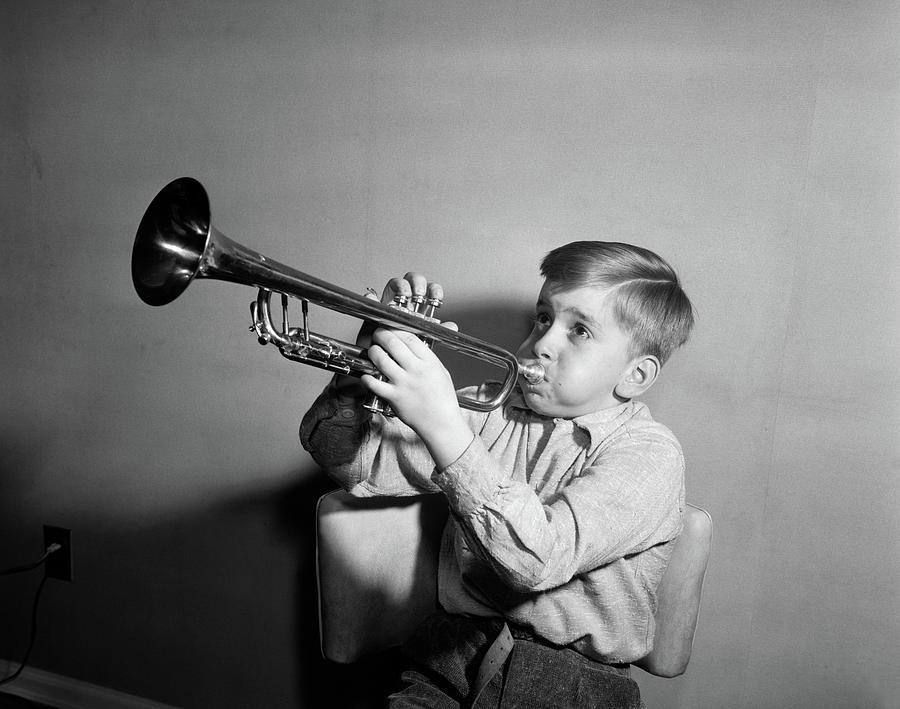This black-and-white photograph captures a young boy deeply engrossed in playing the trumpet, likely from the 1950s or 60s, given the style of his haircut and clothing. He's seated in a white cushioned chair, wearing light-colored, buttoned-up cotton shirt paired with dark, wool-like pants, and a belt that's partially hanging down in front of him. His cheeks are puffed out, indicating he is blowing forcefully into the trumpet, which he holds with his right hand on the keys and his left hand supporting the instrument from below. The trumpet points upward at about a 30-degree angle. He gazes intently towards the left upper part of the frame, focused completely on his performance. The background features a gray wall, white molding at the base, and an electrical socket with two plugs to his right, adding to the vintage feel of the scene.